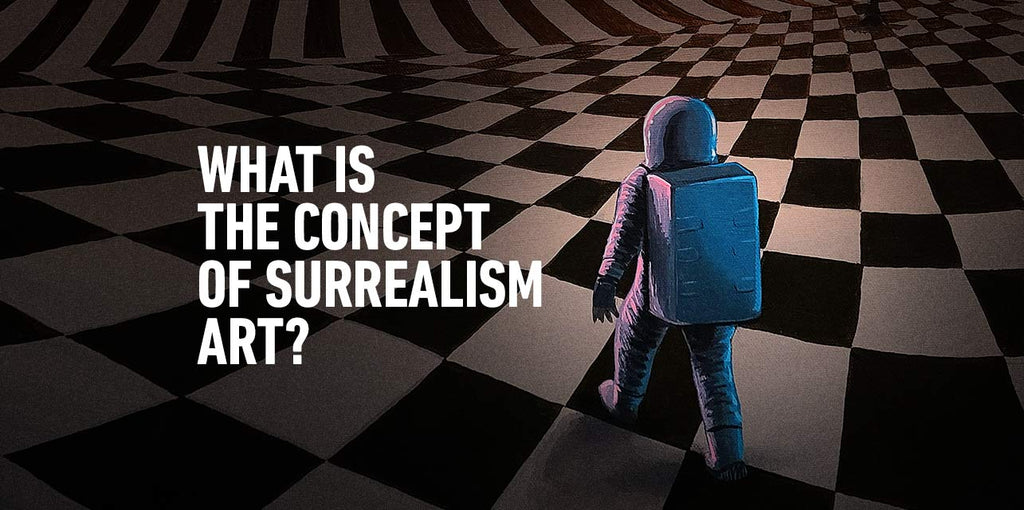The image is a digitally rendered graphic likely created for a presentation or advertisement. Dominating the left side of the background is large, bold white text in all capital letters that reads, "What is the concept of Surrealism in Art?" The text is staggered across four lines, with the question mark at the end, situated about halfway down the image. This inquiry into surrealism is visually supported by the scene on the right: an astronaut, clad in a detailed white spacesuit complete with a helmet, gloves, boots, and a backpack, walks away from the viewer. The astronaut is portrayed as if floating or stepping across a black-and-white checkerboard floor, which starts flat and morphs into a wave-like pattern before tapering off into stripes in the distance. The illusionary and distorted perspective of the floor enhances the surreal quality of the composition, inviting viewers to ponder the intended artistic message.